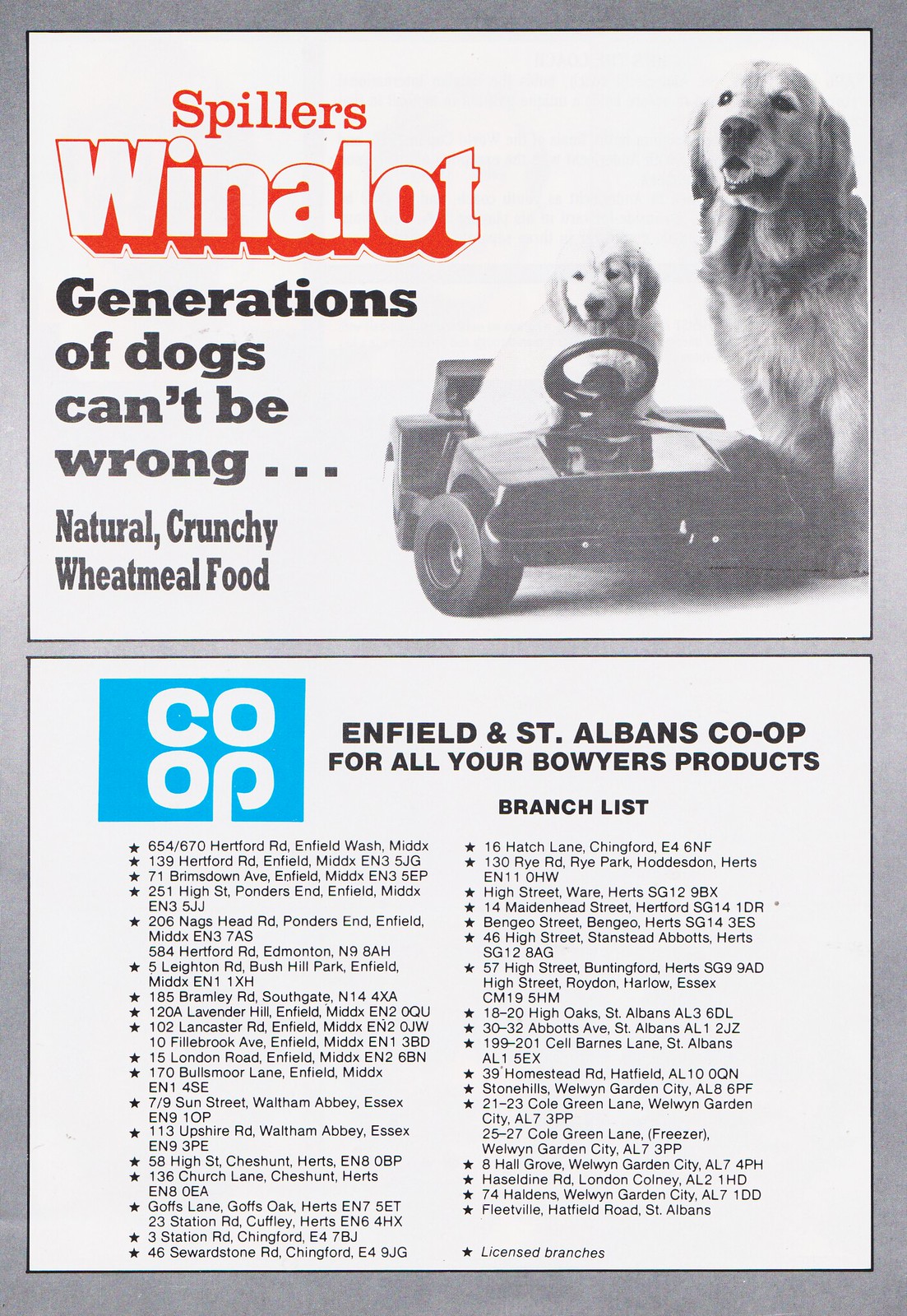This black and white image contains two distinct advertisements, likely from a magazine or pamphlet. The upper half showcases an ad for Spillers dog food, featuring an adult golden retriever and a puppy, with the latter appearing to sit in a toy car as if driving it. The prominent caption in red reads "Spillers win a lot," followed by a black-lettered slogan stating, "Generations of dogs can't be wrong. Natural, crunchy, wheatmeal food."

The lower half of the page displays another advertisement with a blue square containing white letters that spell out "C-O-O-P". In black text next to it, it says "Enfield and St. Albans CO-OP for all your Bauer's products." Below this, there are two columns filled with bullet-pointed information regarding various branches. The entire image is bordered by a gray frame.